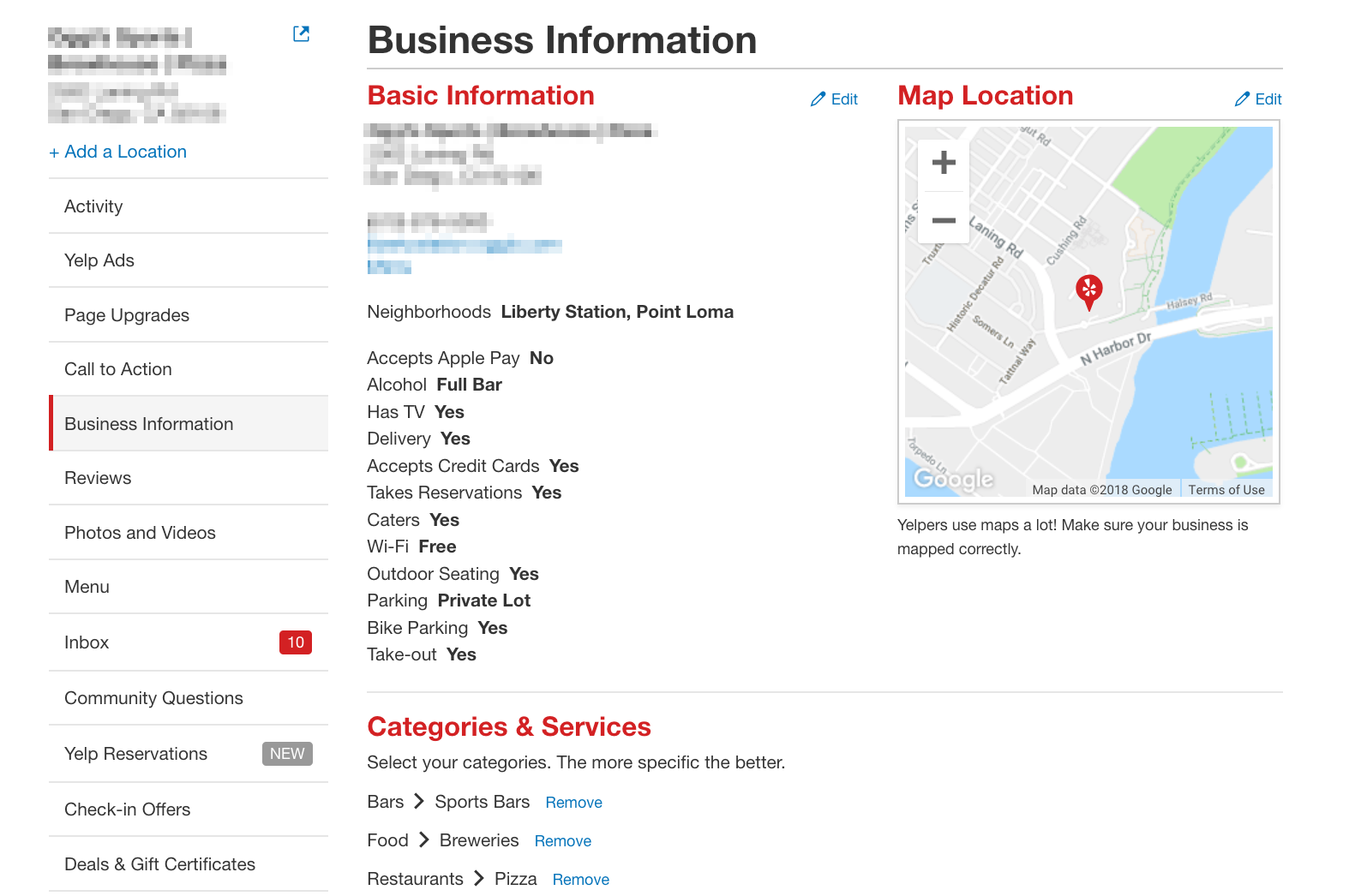The image displays a detailed map on the right side, showcasing a city situated along the edge of a body of water, with the water on the right and the land on the left. A notable feature on the map is a red label marking a specific location in the middle. 

In the center of the image, there is comprehensive business information for a store, outlining its description and address. The listed services include an alcohol bar, TV, delivery, acceptance of credit cards, and free Wi-Fi.

On the left side, there's a list of clickable links for various sections. These sections, from top to bottom, include: Activity, Yelp Ads, Page Upgrades, Call to Action, Business Information, Reviews, Photos and Videos, Menu, Inbox, Community Questions, Yelp Reservations, Check-In Offers, and Deals and Gift Certificates located at the bottom left corner. 

The entire page is set against an all-white background.